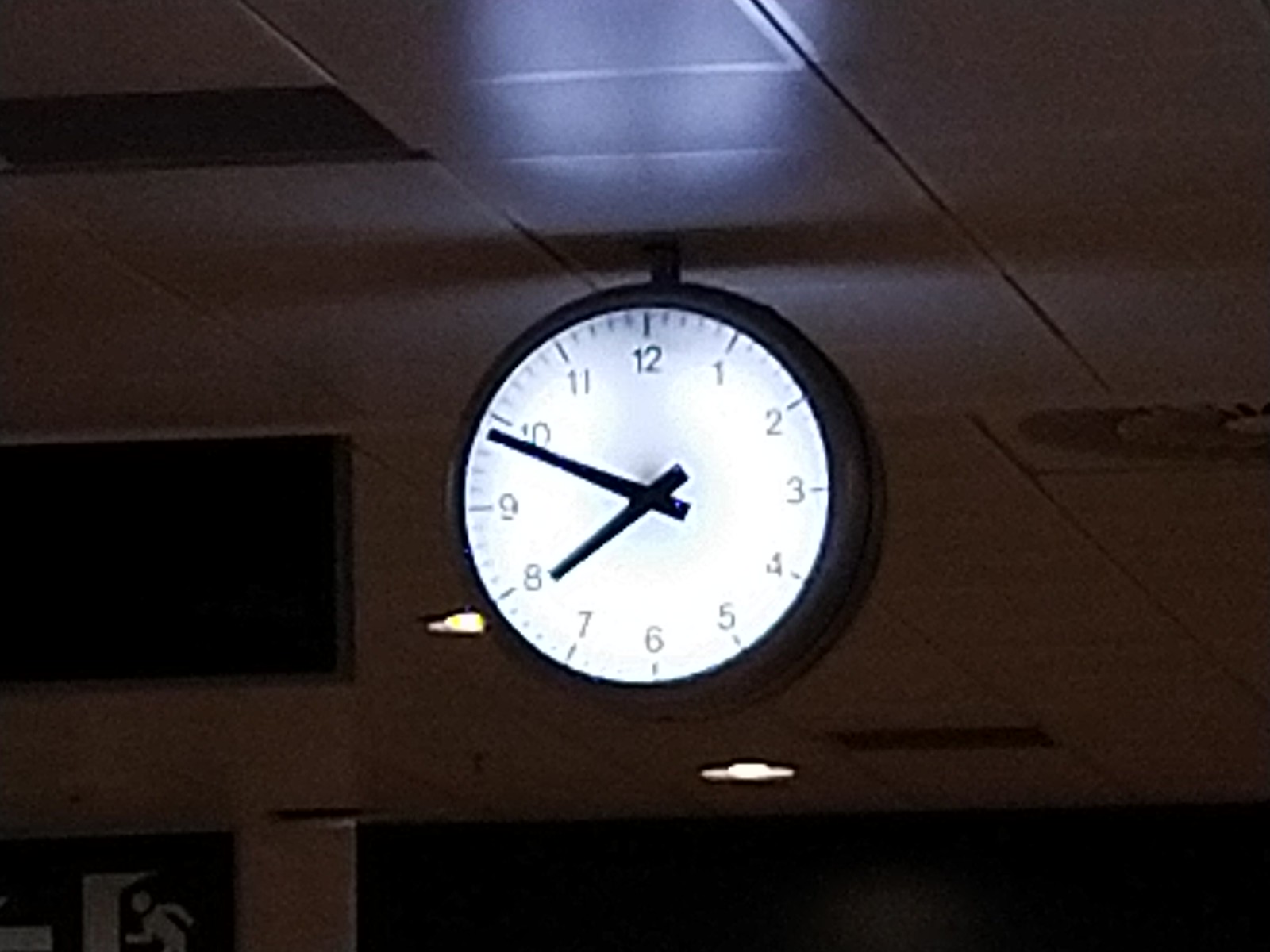The image features a prominently displayed, illuminated analog clock affixed to a drop tile ceiling, likely in a public building setting. The round clock has a white face featuring standard numbers from 1 to 12, small divots for precise time reading, black hands, and a black border. Currently, the time shown is 7:49, with the hour hand just before the 8 and the minute hand just before the 10. The clock's face is illuminated, casting a subtle light that reflects slightly on the semi-shiny ceiling tiles above.

The clock appears to be hanging slightly apart from the ceiling structure, suggesting it may be attached to an upper frame or positioned between ceiling panels. Behind the clock, there's a brown blur, possibly indicative of wooden walls or dividers, hinting that the photo may have been taken in a sectioned-off area like booths in a restaurant. The image overall is dark, but some elements are visible due to the self-illumination feature of the clock. In the lower left corner, there is a sign showing a figure exiting through a door, adding to the public atmosphere. Additionally, a couple of light fixtures around the clock are on, partially lighting up the scene but contributing to the overall dim ambiance.